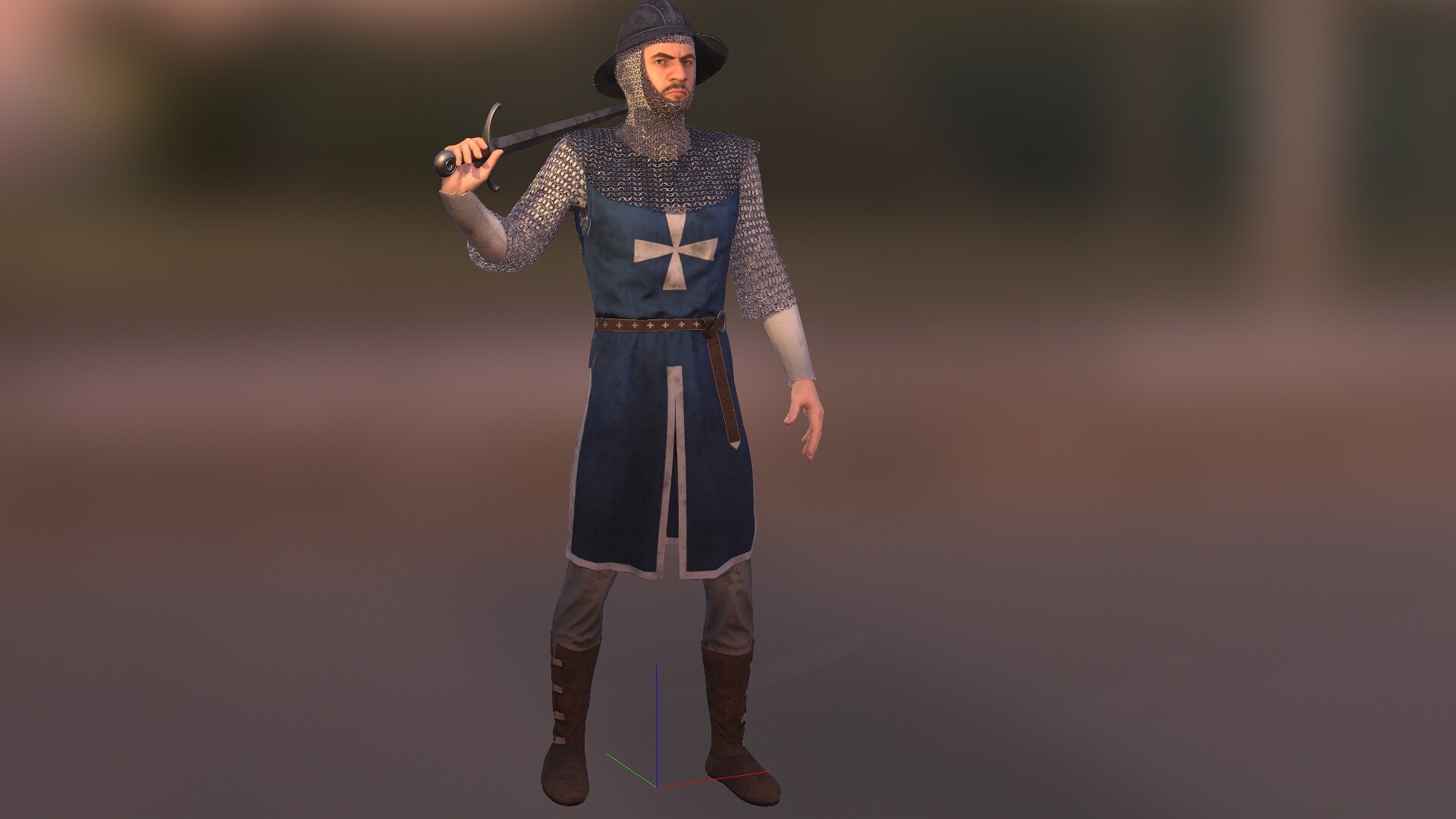The image is a detailed, horizontal, rectangular drawing, similar to what you might see in a video game. The background is heavily blurred, featuring a mix of plum and maroon hues that are indistinct, almost as if the scenery hasn't fully rendered. The sole figure in the foreground is a male character, resembling a knight from medieval times. He stands wearing a rounded, black hat with a large brim, and his face is framed by chainmail that covers his head and neck. He sports brown, arched eyebrows, a brown beard, and a matching mustache, with a very serious or intense expression.

The character is clad in a jade or navy-colored robe that features a prominent silver or gray cross on the front, and the border of the tunic matches the color of the cross. Underneath, he wears a long-sleeved gray undershirt and gray pants. He is adorned in traditional medieval chainmail armor. His feet are shod in brown, knee-high boots made of a suede or leather material. The knight is holding a sword with his right hand, laying it across his shoulder in a display of readiness.